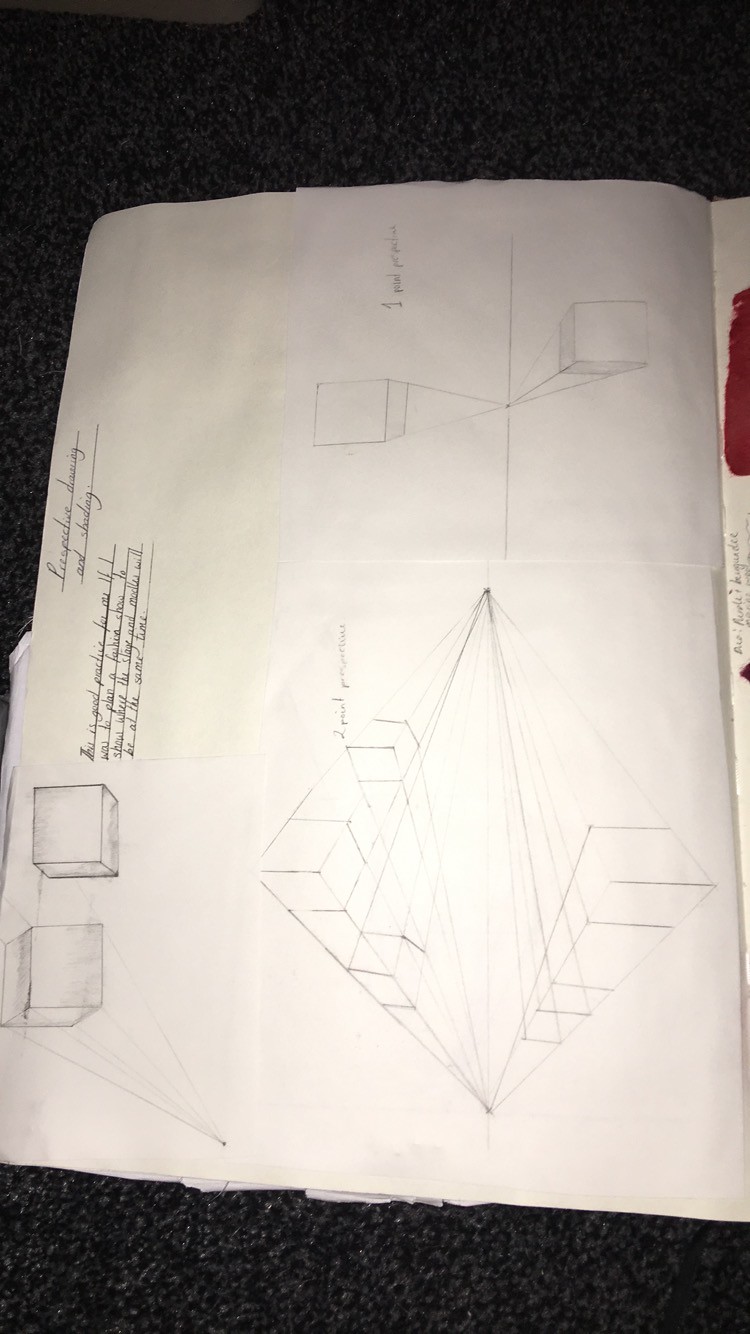An open notebook is spread across a table, revealing intricate pencil sketches and handwritten notes. On the left page, multiple 3D drawings of squares and lines fill the space, accompanied by annotations. The words "perspective drawing and shading" are prominently written, indicating the focus of the sketches. One detailed design features a diamond shape, labeled "two-point perspective," with a simpler "one-point perspective" drawing above it. Below these, a set of four drawn lines carries a note that reads, "This is good practice for me if I was to plan a fashion show to show where the stage and models will be at the same time." A crease divides the notebook, with the right side partially visible. Here, a small burgundy splotch contrasts against the page. Nearby, handwritten cursive notes in purple and burgundy ink add a touch of personalized detail.